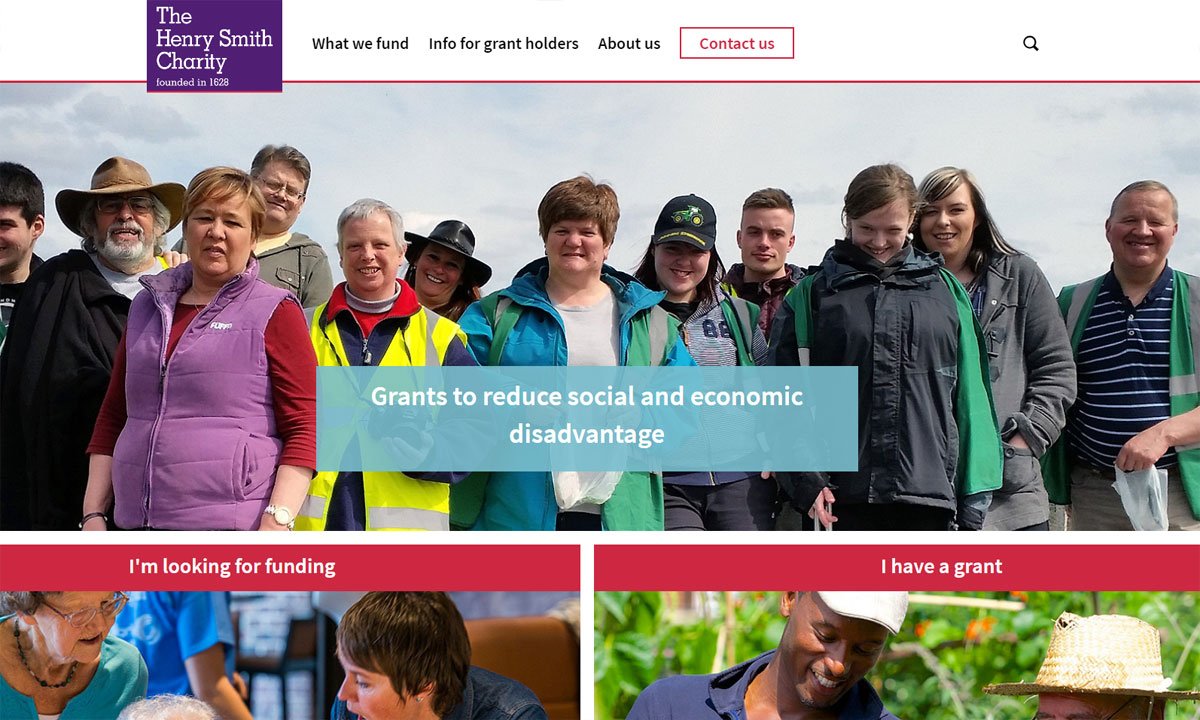This image showcases the homepage of the Henry Smith Charity website, which proudly states its founding year, 1628. On the left-hand sidebar, the menu options include "What We Fund," "Info for Grant Holders," "About Us," and a prominent "Contact Us" button. Below the menu, a vibrant banner features a photograph of a diverse group of people, mostly women, all wearing coats and smiling. Superimposed on this image with a translucent blue background is the text "Grants to reduce social and economic disadvantages." Directly beneath the banner are two distinct sections: one labelled "I am looking for funding" on the left, and the other "I have a grant" on the right. An additional image is visible below these sections, further illustrating the website's layout and design.